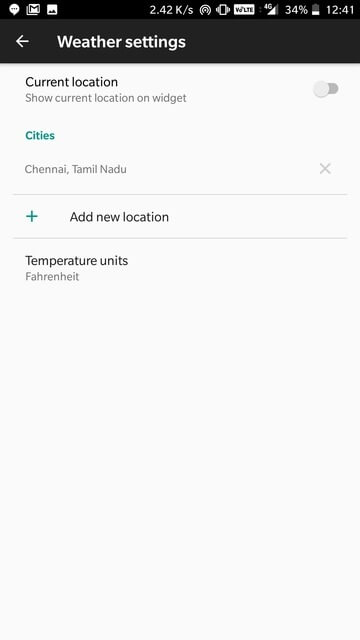This image shows a screenshot taken from a smartphone, focusing on the "Weather Settings" screen. 

At the top of the screen, there's a large black rectangle with a white arrow pointing to the right, accompanied by the text "Weather Settings." Positioned on the left side of this rectangle are three icons, followed by the text "2.42K/S," and four more icons after that. Moving to the right, it displays the battery percentage as "34%" and the current time as "12:41."

The bottom portion of the screen is a very faint gray, almost white. At the top of this section, the text reads "Current Location," followed by an option "Show current location on widget" with a slider switch that is currently in the 'off' position.

Below this, in blue text, is the heading "Cities," with the location "Chennai, Tamil Nadu" listed underneath in gray text. Next to this row, on the far right, there's a gray 'X' icon. Below it, a teal plus sign is shown with the text "Add new location."

Further down, in black text, it reads "Temperature Units," and underneath, in gray text, the unit "Fahrenheit" is displayed.